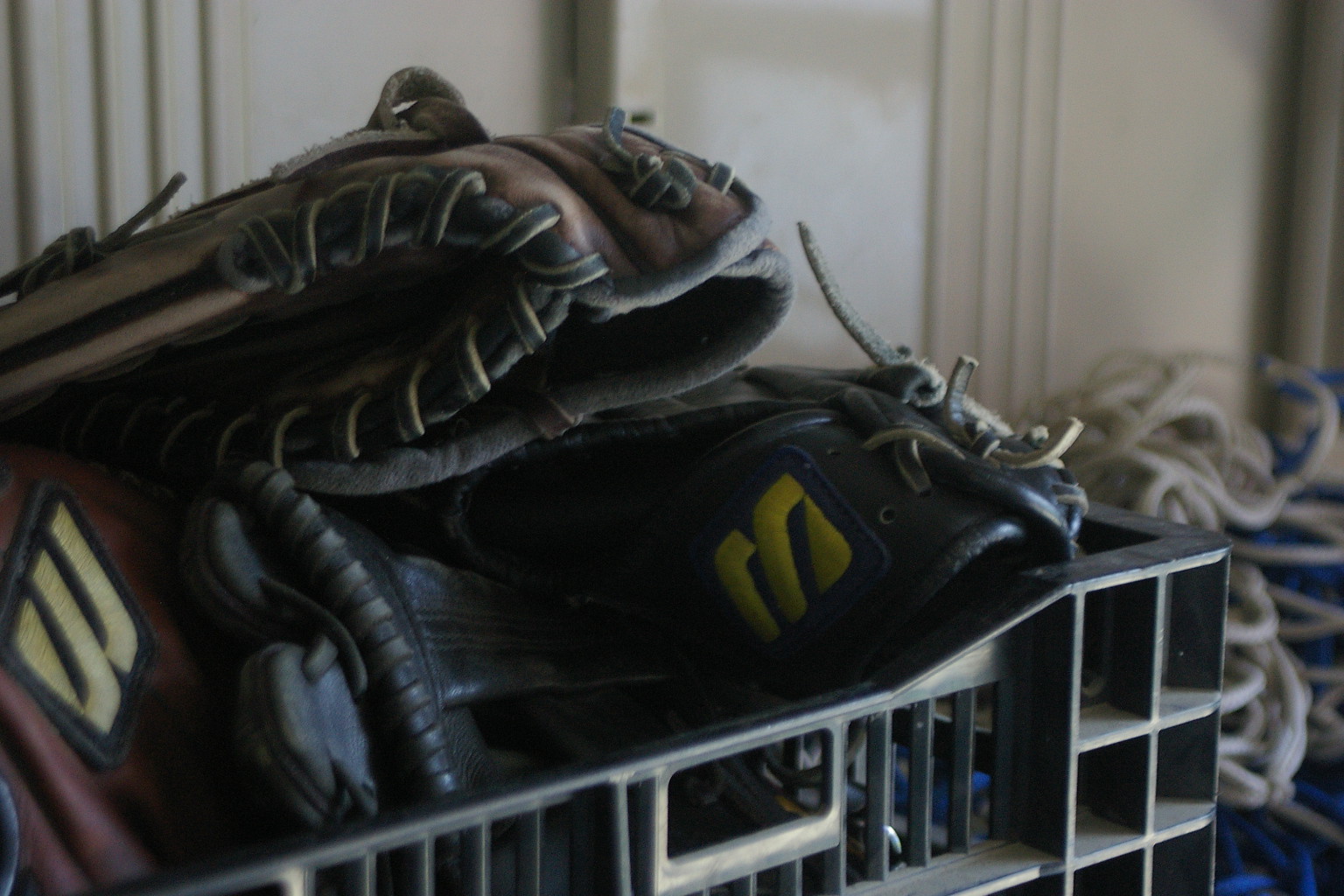This somewhat dark photograph features a large black plastic milk crate in the foreground, filled with a haphazard assortment of well-used baseball gloves in various sizes. The gloves are predominantly tan, red, and black, with visible stitching and two prominently displaying Wilson logos. Behind the crate is a white wall with visible molding and shapes. To the right of the crate, a pile of loose, thick shoelaces, or possibly nylon ropes in tan, white, and blue, is partially visible. The gloves and crate are sharply focused, contrasting with the slightly blurry background and ropes. The scene captures a sense of organized chaos, emphasizing the varied yet familiar elements of baseball gear.